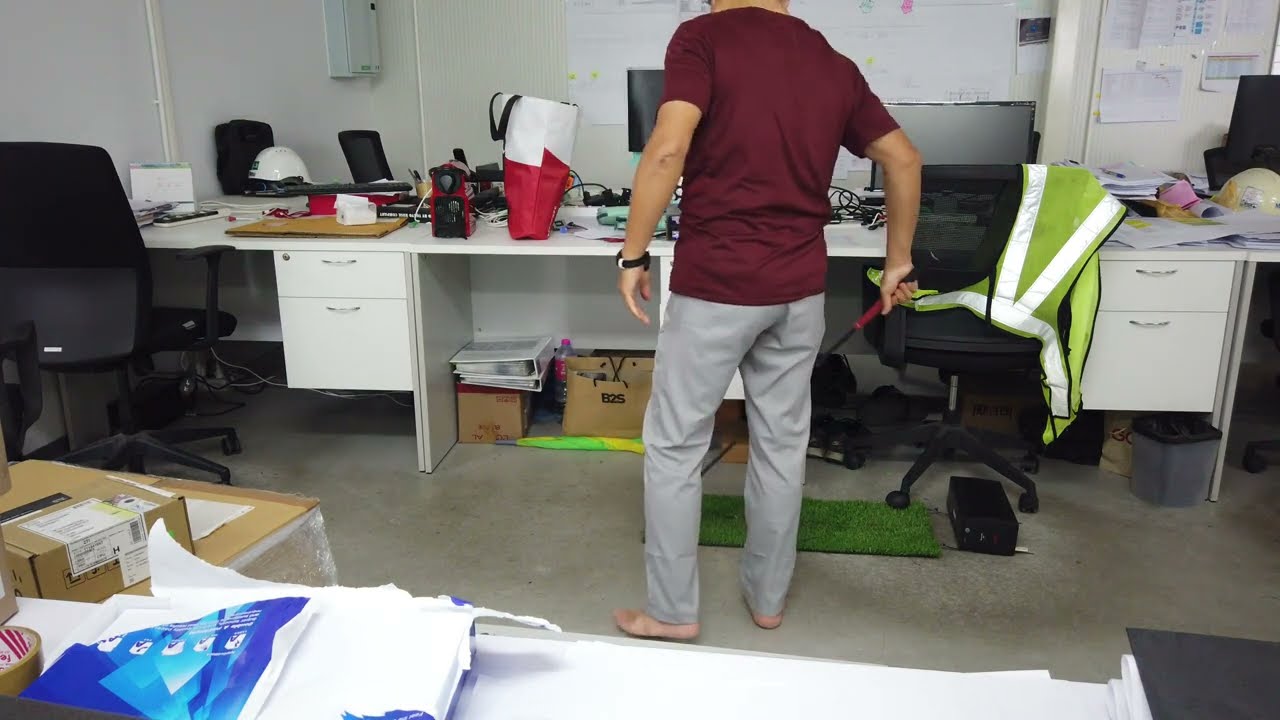In the center of the image is a barefoot man wearing khaki pants and a burgundy short-sleeve shirt, with his back towards the camera and holding a golf putter. He stands on a green mat resembling an office putting green, positioned near a black office chair that has a yellow neon safety vest draped over it. The setting appears to be an office or study room with white walls and is highly cluttered. Along the wall in front of him are papers and calendars. There are three white desks lined up against this wall, each cluttered with various items. The desk to the left has technical devices that might be speakers, and in front of it is a black office chair. The man stands facing the center desk, which hosts a red container, a computer monitor, and some boxes underneath. To his right is another identical white desk, this one with books and a pink item on its surface. In the foreground is a white table with an open pack of bulk paper in blue wrapping, and to the very left side are boxes with labels, presumably ready for shipping. The room features a grayish-white linoleum floor, adding to the chaotic yet functional ambiance of the space.